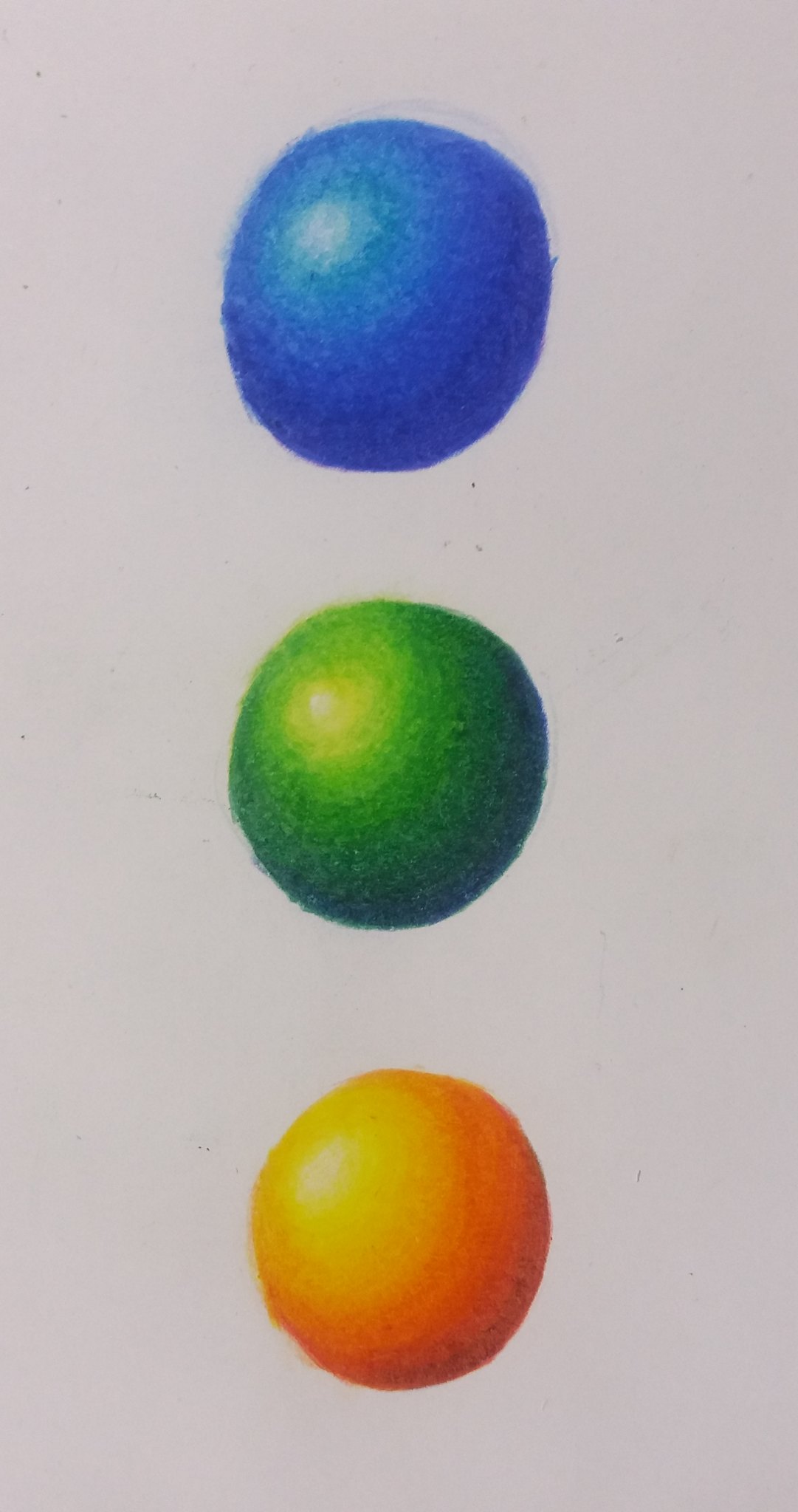The image features three horizontally stacked circles set against an off-white, light gray backdrop. The top circle is dark blue with a small tinge of white located towards its middle left area, giving it a part-reflective quality. Below it, separated yet perfectly aligned, is a rich green circle that lightens towards the middle, transitioning to an almost yellow hue. The bottom circle, similar in size, is a darker orange that gradually becomes a lighter orange, fading into a light yellow with a small, white central spot. The arrangement of these circles resembles a traffic light but employs different colors. The watercolor-like texture of the circles gives them a soft, fuzzy appearance overlapping slightly but not touching one another. Each circle features a subtle gradient and reflective spots, enhancing the illusion of volume and light reflection.